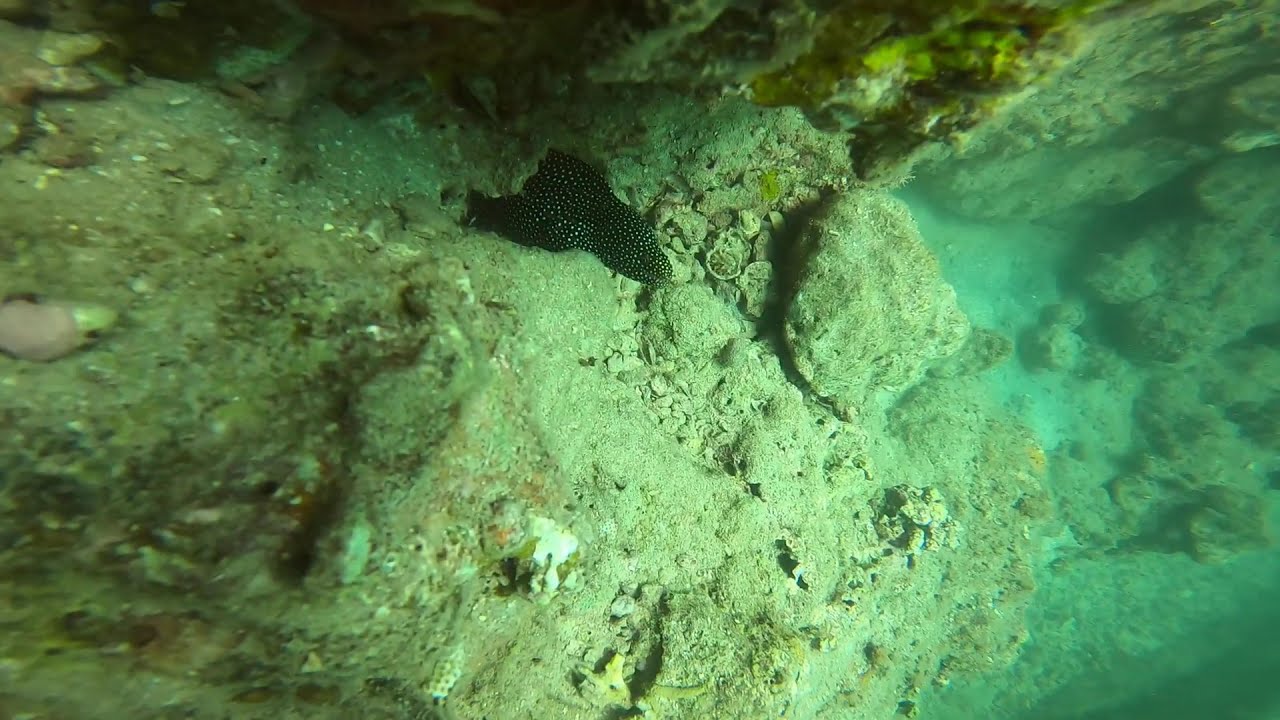This underwater photograph depicts a seabed scene bathed in hues of greenish-blue. Central to the image is a prominent black fish adorned with numerous white dots, resting on a sandy and rocky ocean floor. Jagged rock formations dominate the area, forming ledges that cascade over deeper sections where the water appears slightly cloudier and more bluish-green. Among the rock formations, patches of algae are visible, contributing to the natural color palette of blues, greens, and yellows. To the middle and far left, a pinkish object, possibly an odd-colored rock or another sea creature, intrigues the viewer. Scattered across the sandy floor near the black fish are several seashells, some partially filled with sand, and a noticeable white shell gleams from beneath the sediment. The setting conveys a tranquil yet mysterious underwater world rich with texture and life.